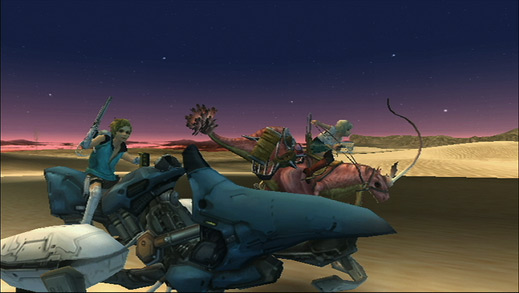In this illustration, likely derived from an online video game, a dynamic female character with flowing blonde hair is depicted in the heat of battle. She is clad in a striking blue outfit with long white boots and brandishes a gleaming sword. The formidable heroine is astride a mechanical contraption that intriguingly blends the elements of a motorbike and a dragon. She engages an indefinable, smooth-skinned creature, which remains enigmatic with no recognizable animal features.

To the left of this valiant figure lies an enigmatic white, egg-shaped object, adding an element of curiosity to the scene. In the backdrop, a fantastical, silvery-white creature rides a creature resembling a pink dinosaur, further enhancing the surreal atmosphere. The environment is set amidst a sandy terrain under a mysterious purple sky, creating a vivid and immersive fantasy world.